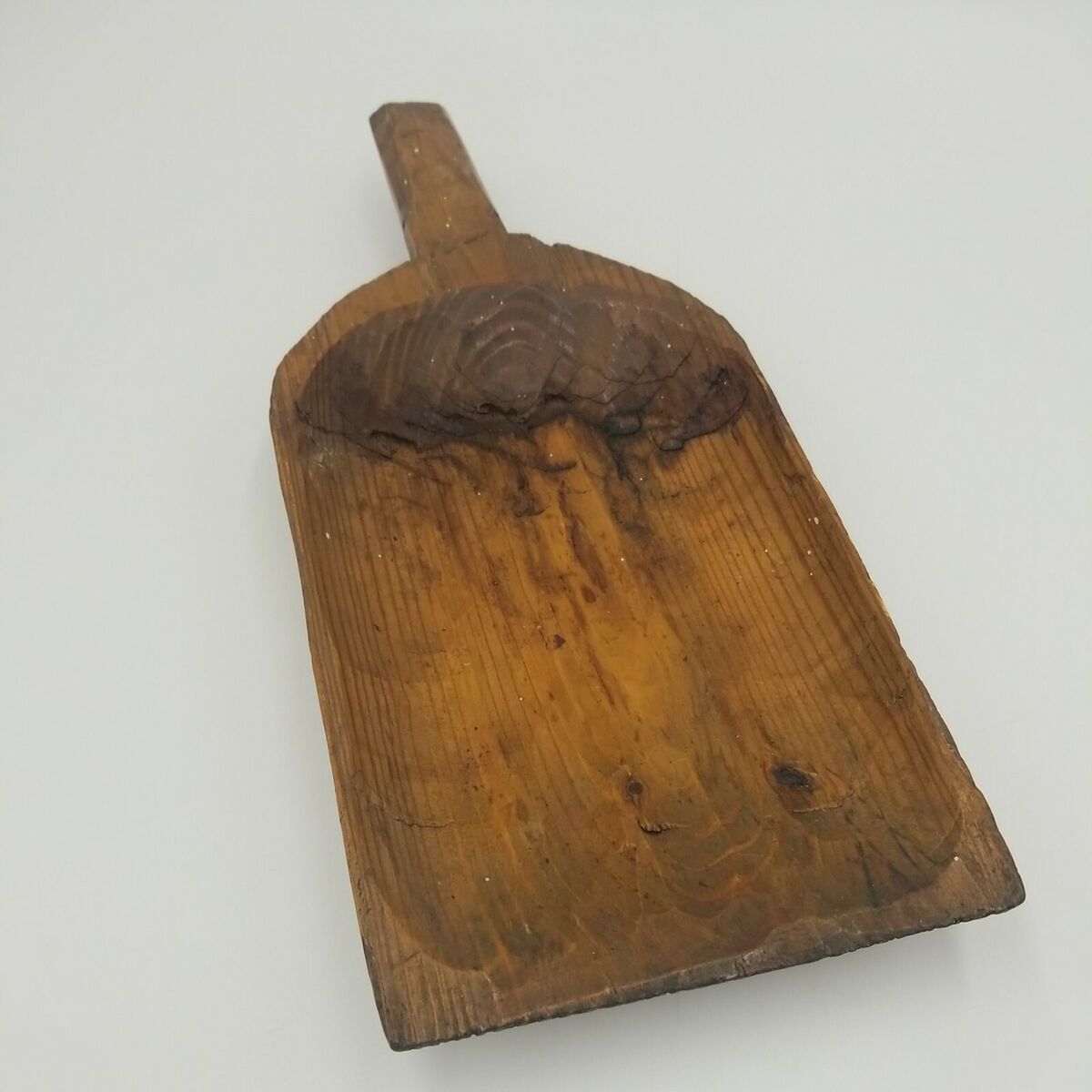The image features a well-used wooden paddle set against a cream-colored background. The photograph, taken from a slightly diagonal, bird's-eye view, captures the paddle in portrait orientation. The paddle is fairly worn, with visible discoloration and signs of heavy use. It appears carved with marks along its light orangey-yellow-brown surface, transitioning to a darker brown nearer the short, nub-like handle. The wood has a flat surface with slight flaring at the sides, ending in a blunt edge. The top of the paddle has noticeable wood knots and a bulging, oval-shaped dark mass that appears rigid and irregular. This paddle resembles a pizza peel, used for placing pizzas in the oven and retrieving them, suggesting it has been exposed to significant heat.